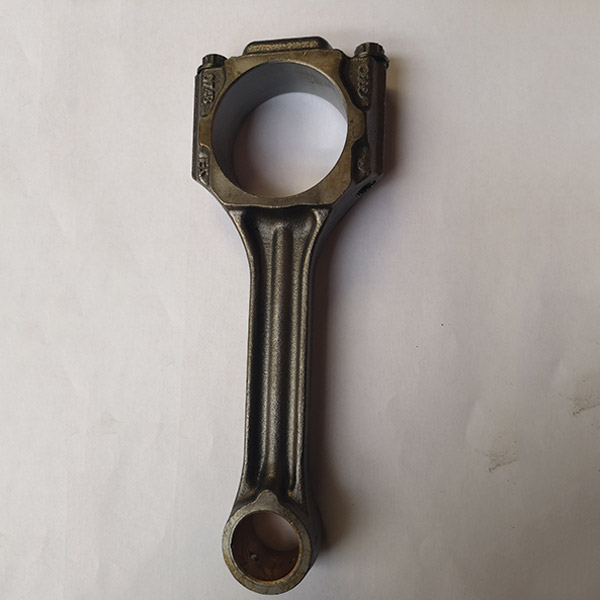This is a detailed close-up image of a metallic device, centrally positioned within a wide vertical rectangular frame against a light gray background. The device, predominantly brown in color, exhibits signs of wear, suggesting it's a vintage or antique piece. Its construction includes several distinctive components: the bottom features a circular opening, indicative of a connecting point for mechanical parts. Extending upward from this circle is a thin vertical rectangular shaft with a central ridge, which leads to a square section. Inside the square, there is another circular opening, reinforced with patterns and designs along its sides. Additionally, the top center of the square has notable flat, tall ridges, which are also present on its top right and left corners. The entire piece, resembling a component of a car engine such as a connecting rod, seems to be held together by large bolts, adding to its rugged, functional appearance.